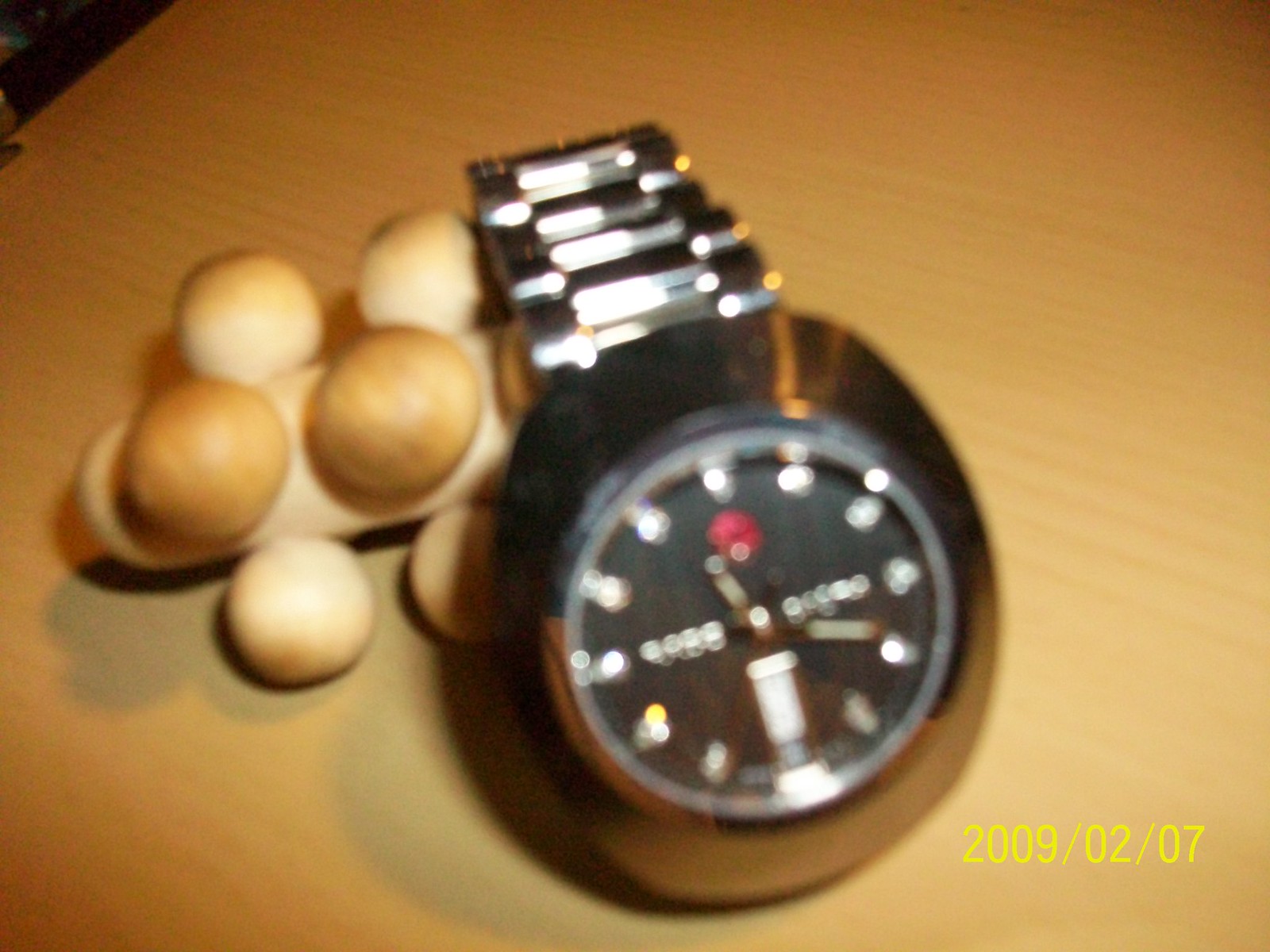This photograph, taken on 2009-02-07, shows a slightly blurry image of a watch resting on a tan and medium brown-colored cylindrical massager with nubs around its edges. The tabletop it sits on is a light blonde wood with visible grains, somewhat plain, without any darker linings or rustic features. The watch itself features a stainless steel band and a metallic black outer shell around its face, which is black with silver markings. A small red dot is positioned below where the 12 would be, and there are white dots encircling the face instead of numbers. In the photo's background, towards the upper left, the table's edge and a black object are faintly visible.